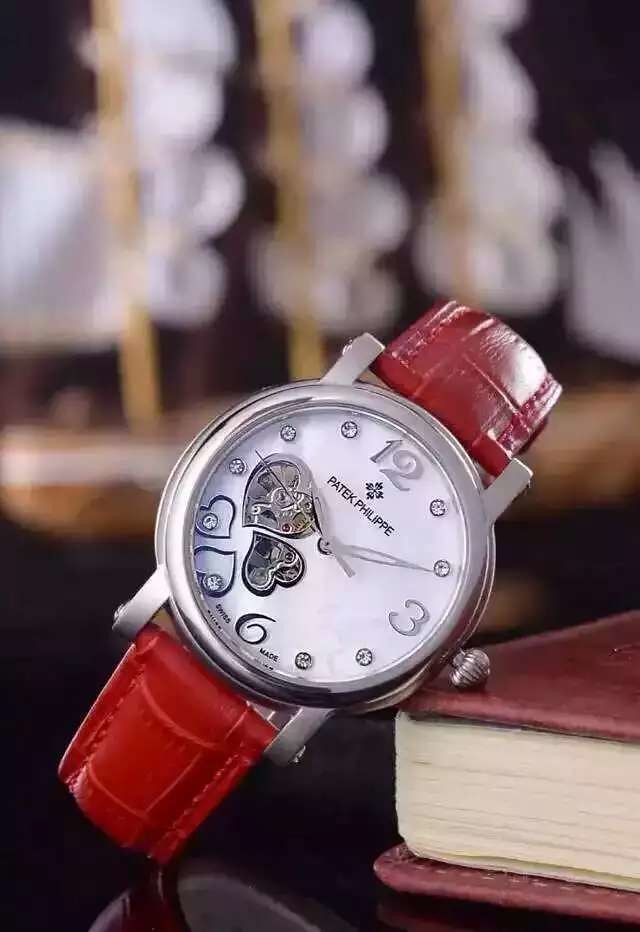A detailed wristwatch is prominently displayed, tilted to the right for an optimal view. The watch boasts a vibrant deep red, almost orangish band, which is complemented by a sleek silver edge encircling the face. The band is secured with silver connectors, adding to its elegant appearance. Inside the face, the numbers 12, 3, and 6 are marked in silver, elegantly standing out. The centerpiece features two delicate heart designs, accompanied by silver minute, second, and hour hands. The watch face is further adorned with intricate diamond-like details representing the other numbers, and additional decorative filigree hearts. The background is artistically blurred, leaving it indistinguishable and drawing all focus to the timepiece. The silver winding crown is visible, indicating the watch's orientation. The wristwatch rests atop a corner of a reddish-brown leather-bound book, which adds a classic touch to the composition. The book appears thick, with its white pages slightly fanned out, revealing a textured surface. The side of the book's pages is partially visible, showcasing fine details in the craftsmanship.